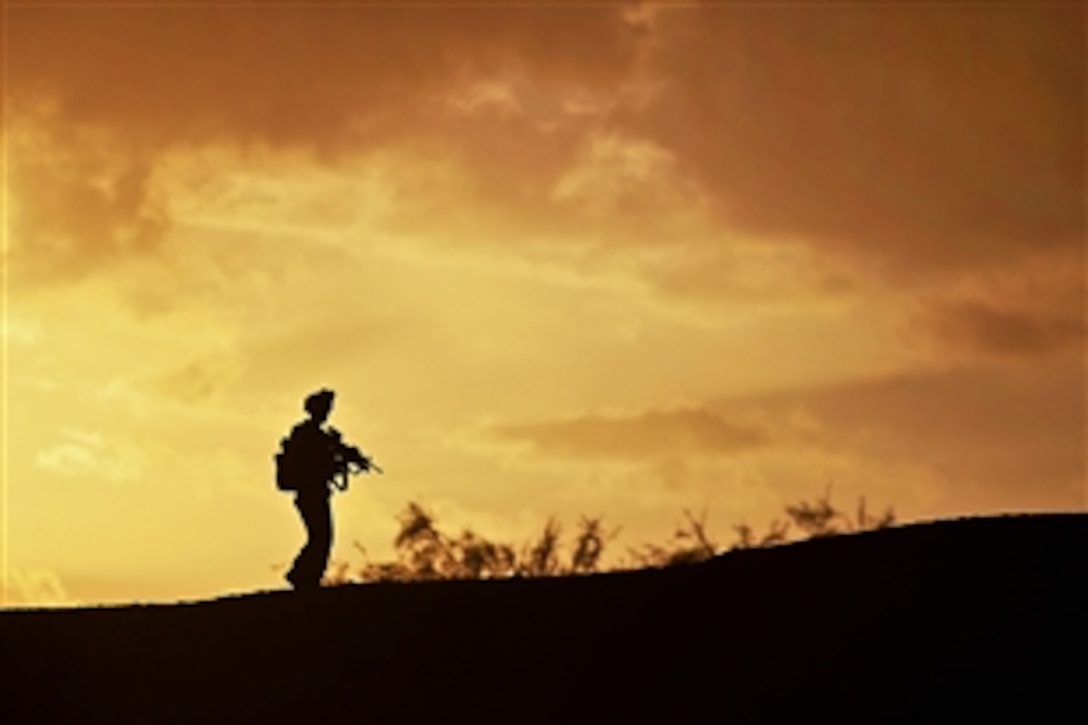In this outdoor image, a blurry and somewhat ambiguous scene is captured, possibly at sunset or during a smoky event such as a fire or even a war. The sky dominates the background with a blend of vivid colors—deep orange, rich red, and bright yellow—intermingling, suggesting either the setting sun or distant flames. Along the bottom of the image stretches a dark, brownish-black hill, silhouetted against the vibrant sky. Plant life is faintly visible, adding texture to the scene. A lone figure, likely a man, is silhouetted on the left side of the hill. He appears to be dressed in tactical gear, wearing a helmet and holding a large rifle. A backpack is visible on his back, emphasizing his preparedness. The overall scene is somewhat blurry, lending a sense of mystery and tension, further accentuated by the stark contrasts and dark tones of the ground and sky.